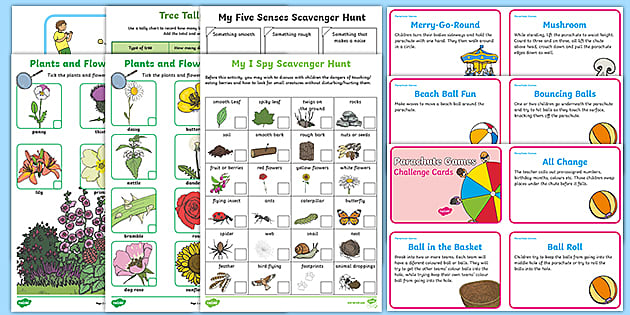The image depicts an expansive, light blue background that showcases a variety of activity pamphlets and cards, primarily related to party and scavenger hunt games, aimed at children. On the far right, there is a stack of red-outlined rectangular cards, each describing different games such as "merry-go-round," "beach ball fun," "ball roll," and "bouncing balls," with accompanying descriptions. The column on the right includes titles like "mushroom" and "bouncing ball," while the left column lists "merry-go-round," "beach ball fun," "parachute games," and "challenge cards." 

On the left side of the image, several overlapping pamphlets detail different scavenger hunts. Visible titles include "My Eye Spies Scavenger Hunt" and "My Five Senses Scavenger Hunt." These pamphlets feature various natural elements like leaves, branches, insects, and rocks, each with checkboxes to mark off found items. Each scavenger hunt seems to focus on outdoor exploration and sensory experiences, such as identifying specific plants, trees, and flowers. The overall scene suggests a vibrant mix of interactive, nature-themed activities designed to engage children in playful and educational pursuits.